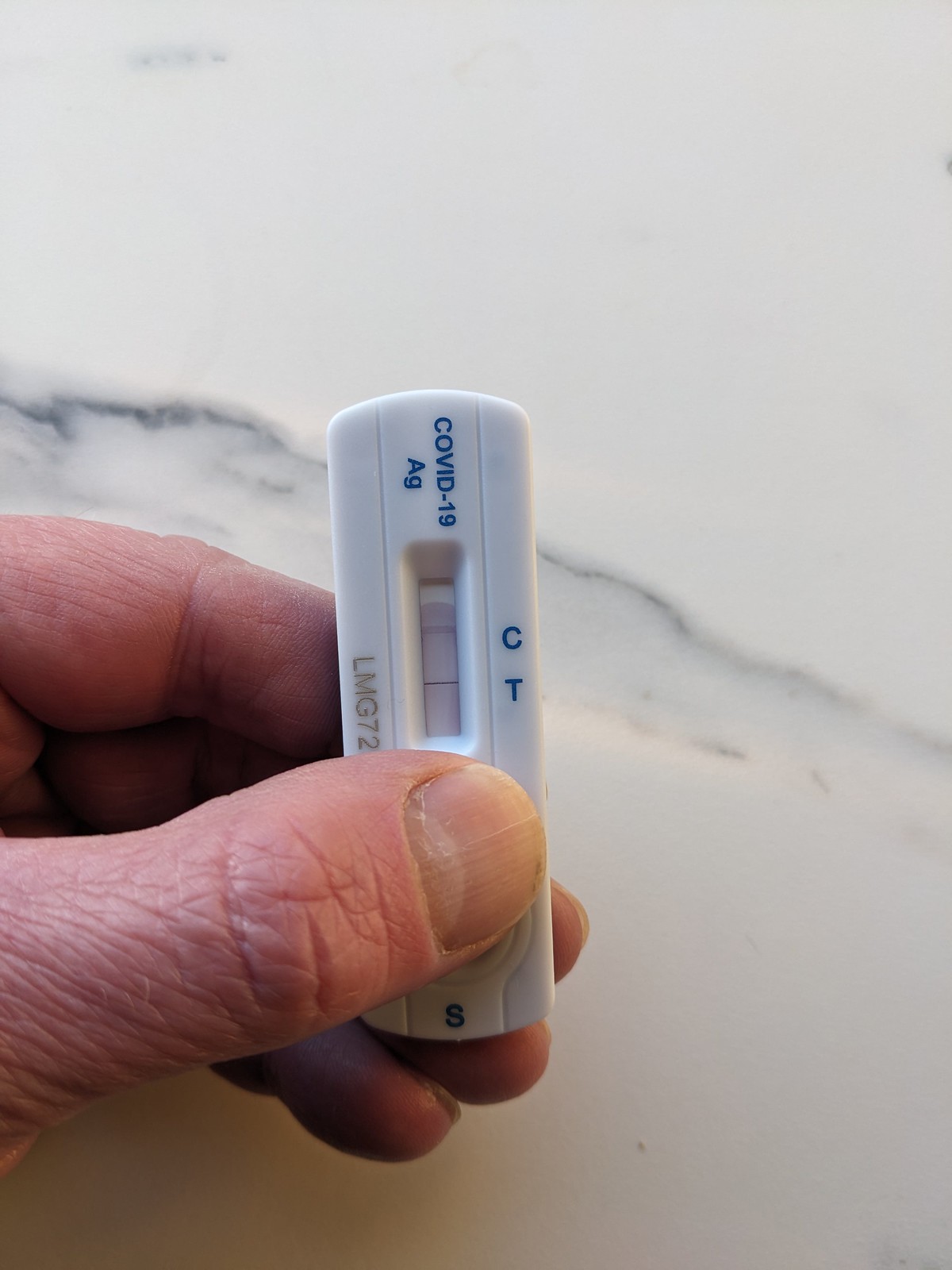A person holds a small, white, rectangular COVID-19 home test kit in their left hand. The kit, made from plastic, features slightly rounded edges. The individual's thumb secures the top of the kit, which is labeled "COVID-19" followed by "AG." Centrally located on the test kit is a small, window-like feature designed to display test results. To the right of this window are the letters "CT," while on the left side, the code "LMG72" is visible. At the very bottom, just below the person's thumb, is the letter "S." The background reveals a marble countertop with noticeable swirling patterns, providing a contrasting backdrop to the white test kit and the person's hand. The image captures the test kit's details and its intended use for at-home COVID-19 testing.